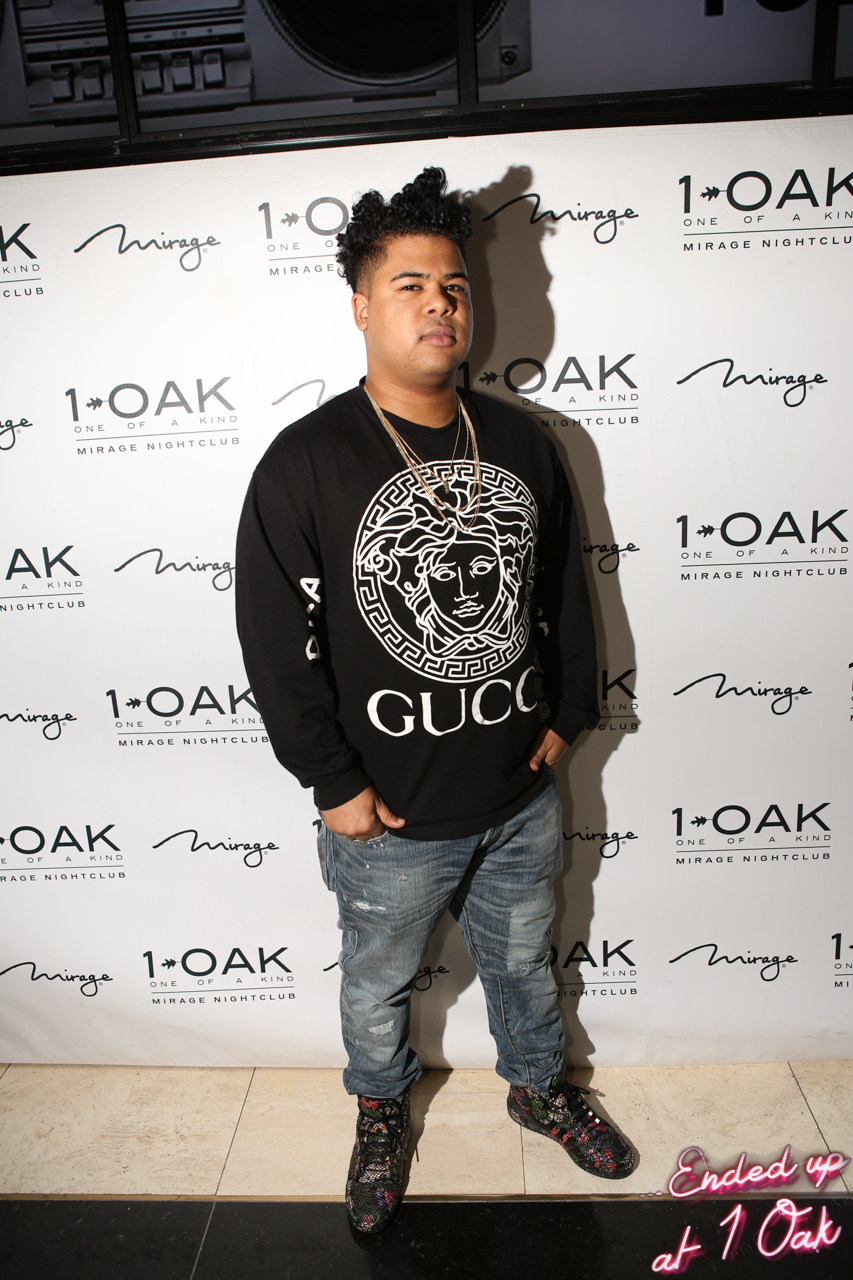The image depicts an African-American gentleman standing indoors, centered in front of a large advertisement billboard for the Mirage Nightclub, prominently featuring the text "One Oak" and "ended up at White Oak" in the bottom right corner in pink. The billboard is predominantly black and white with repeating elements of the Mirage logo. The setting appears to be a nightclub with a multicolored tile floor in shades of black, tan, purple, and blue. 

The man is casually dressed, sporting a black Gucci sweatshirt adorned with a white drawing of a woman's face and the brand name "GUCCI" in large letters beneath it. He wears faded blue jeans and black shoes, and accessorizes with a gold chain around his neck. His hands are casually placed in his pockets. Above the billboard, there appears to be another, partially visible board with some form of radio or music player. The overall color scheme of the image is subdued, primarily black and white with some beige flooring.